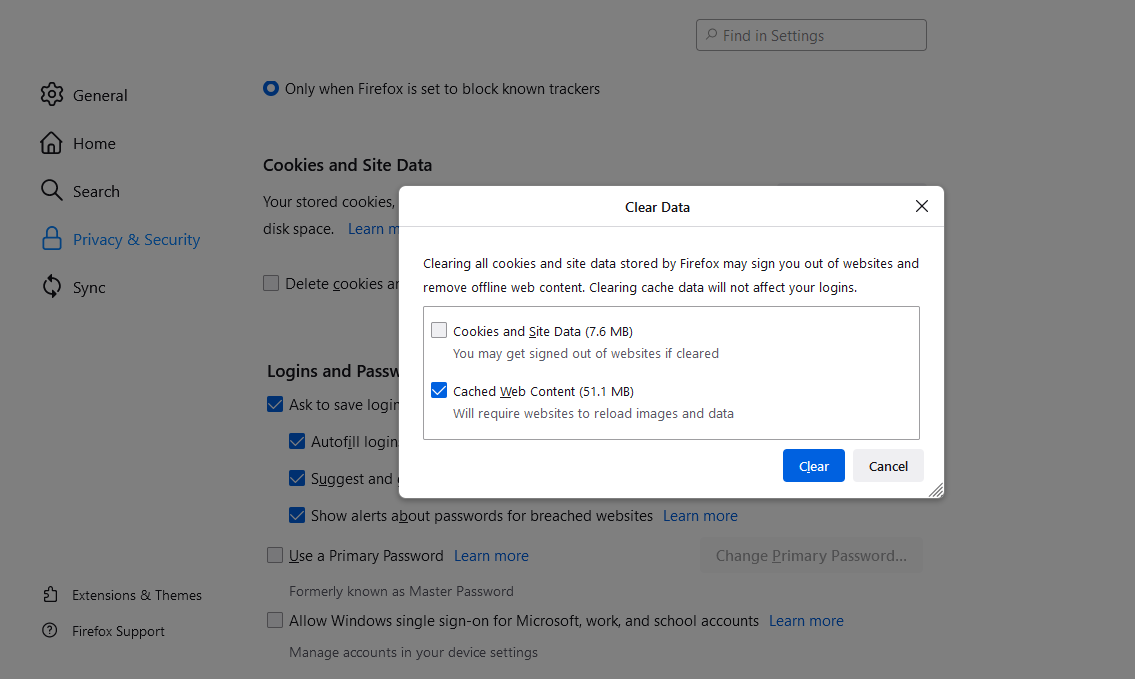The image displays a screenshot of a computer screen, with the main focus on a prominent white pop-up window in the center. The screen's background appears grayed out, indicating it's not the active element. The white pop-up, titled "Clear Data," has an 'X' icon at the top-right corner, which allows users to close the window.

Within the pop-up, there's a message warning users that "clearing all cookies and site data stored by Firefox may sign you out of websites and remove offline web content. Clearing cache data will not affect your logins." Below this warning, another section within the white pop-up window contains two clickable checkboxes.

The first checkbox is labeled "Cookies and Site Data," with "7.6 MB" noted beside it, alongside a clarification that clearing this data may sign users out of websites. The second checkbox, labeled "Cached Web Content," shows "51.1 MB" and explains that clearing it will "require websites to reload images and data." At the bottom of the pop-up, there are two buttons: one for "Clear," to confirm data clearing, and another for "Cancel," to exit without making changes.